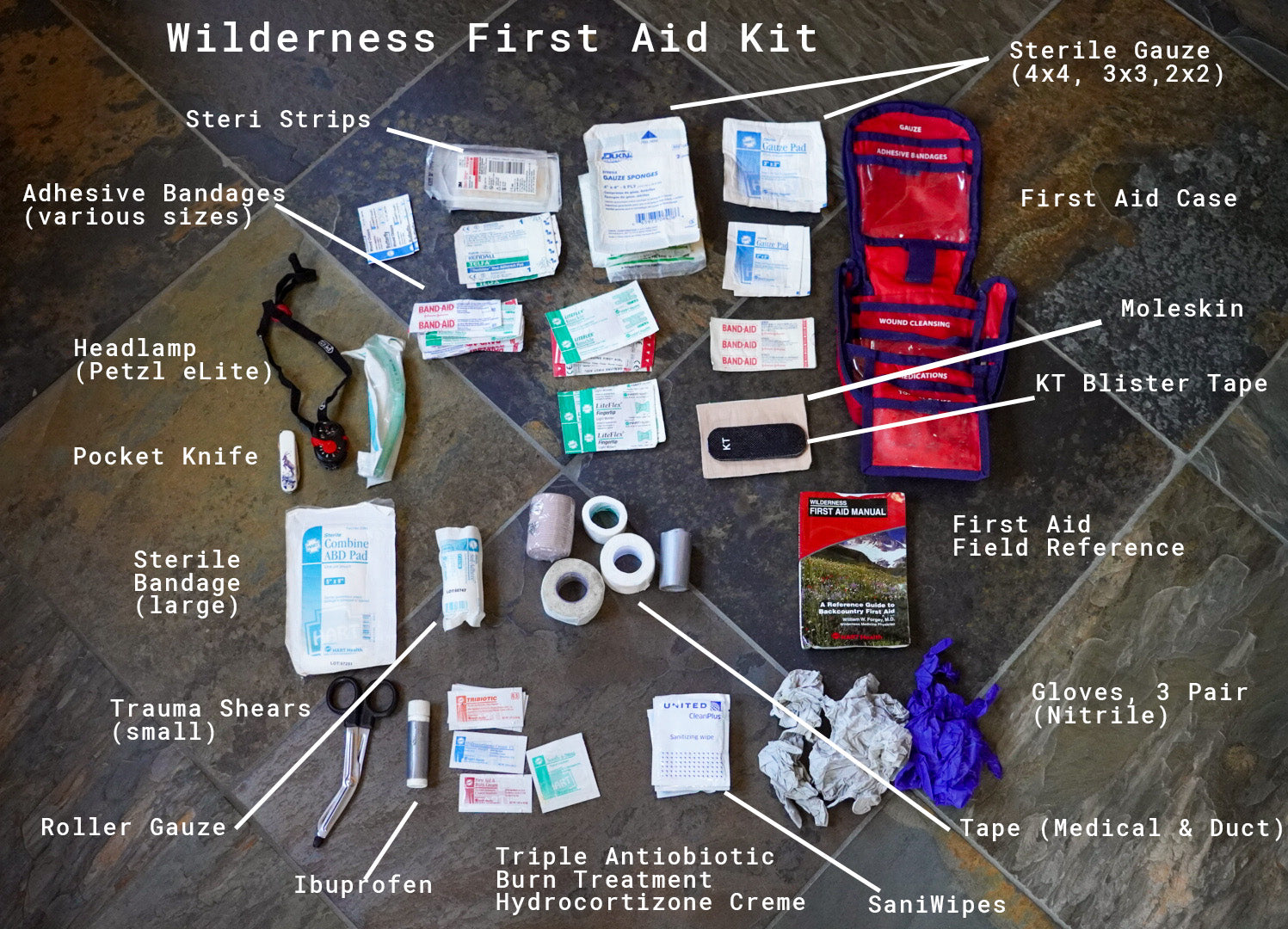This color photograph displays an array of first aid items meticulously labeled with white text and connecting lines, scattered across a brown tiled floor with white grout lines. At the top of the image, in bold white text, it reads "Wilderness First Aid Kit." The background tiles have a yellow-green-gray marble-like pattern. Prominently positioned in the upper right is a red first aid case. The items include steri-strips, adhesive bandages of various sizes, a headlamp, a pocket knife, large sterile bandages, trauma shears, roller gauze, ibuprofen, triple antibiotic and burn treatment hydrocortisone cream, sani-wipes, medical tape alongside duct tape, and three pairs of gloves. Additionally, there's a first aid field reference guide. Trauma shears are located at the bottom left, vinyl gloves at the bottom right, and a small booklet on the right, showcasing a comprehensive Wilderness First Aid Kit.